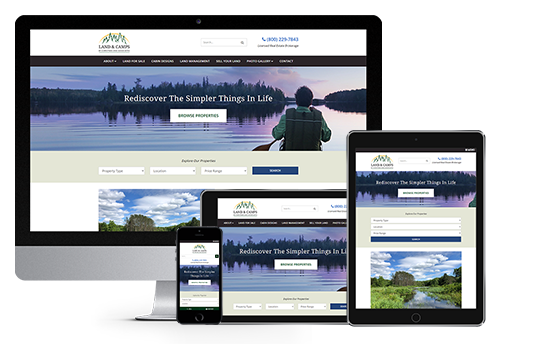The image showcases a website displayed across various Apple devices, including a desktop computer with a large black bezel and a silver stand, an iPad with a black bezel, a smaller smartphone, and another iPad in portrait mode. The website features the title "Land in Canoe" alongside green tree icons, suggesting an outdoor or nature theme. The site includes a blue phone number on the right, and beneath it, a tagline: "Rediscover the simpler things in life." A call-to-action button labeled "Browse Properties" is visible, accompanied by an image of a man in a life vest holding a paddle, seemingly on a lake surrounded by distant trees. Additionally, there is a scenic picture of an outdoor area with clouds, a river, and lush greenery. The resolution is slightly low, making the text and finer details harder to discern.